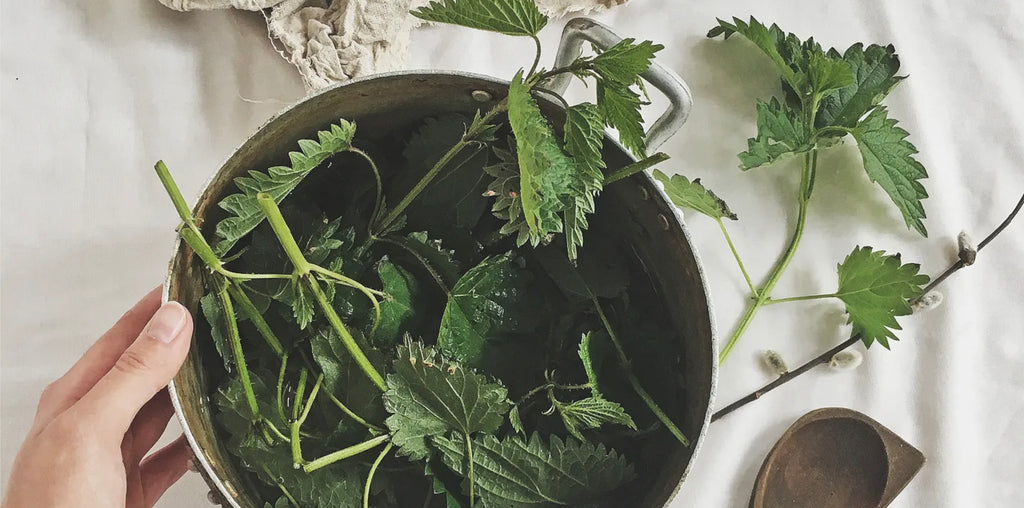In this horizontal color photograph, we are looking down at a silver metal bowl, appearing worn and darkened with age, sitting on a white cloth that covers a table. The bowl is slightly off-center but takes up most of the image, and it contains various rough, dry green leaves still attached to their stems, likely being washed. Some leaves spill out onto the white cloth to the bowl's right. A slightly tan but mostly fair hand, presumably Caucasian, is seen at the upper left, with a thumb and three fingers gripping the bowl. In the lower right of the frame, there is a handcrafted wooden spoon, while in the upper left, a curled-up fabric napkin or towel is visible. The scene is softly illuminated, hinting at ambient light from either a window or room lighting.